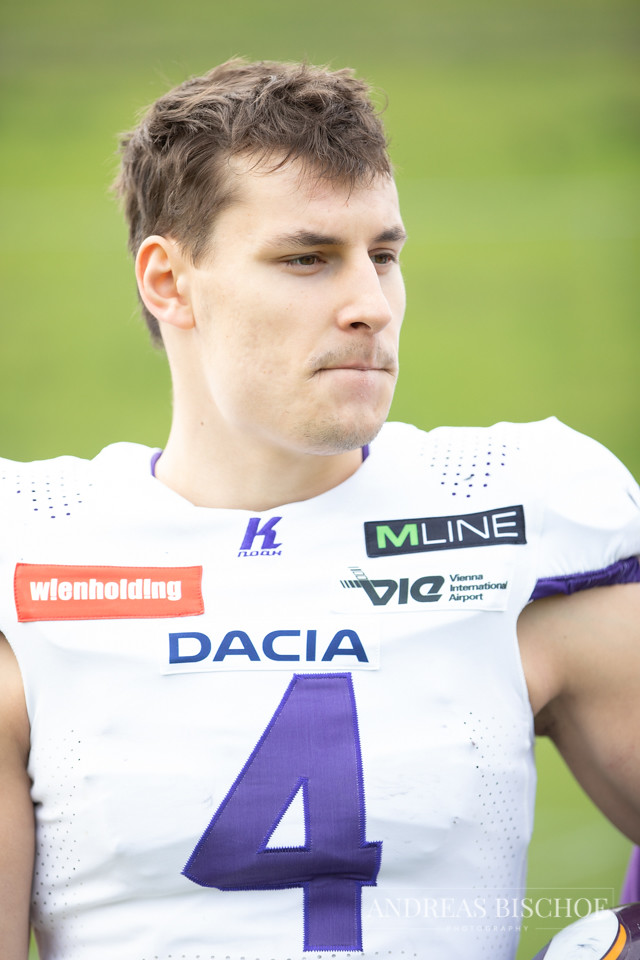In the photograph, a young Caucasian male football player, likely in his 20s or 30s, is seen in a white, sleeveless uniform heavily adorned with sponsor logos, some in English and others in what appears to be German or Swedish. Prominently displayed in purple on his chest is the number 4, with "Dacia" written above it. His logos include "Wienholding" in an orange rectangle on his right shoulder (left in the photo) and "M Line" on his left shoulder (right in the photo) within a black rectangle. The player has short brown hair, light facial hair featuring a slight mustache and goatee, and well-defined muscular arms visible due to the sleeveless design. He's looking off to his left (our right) with pursed lips, suggesting thoughtful contemplation. The background is a blurred green, providing no specific detail. Notably, the bottom right corner bears a hard-to-read watermark in white reading "Andreas Bischoff Photography," blending into his uniform.